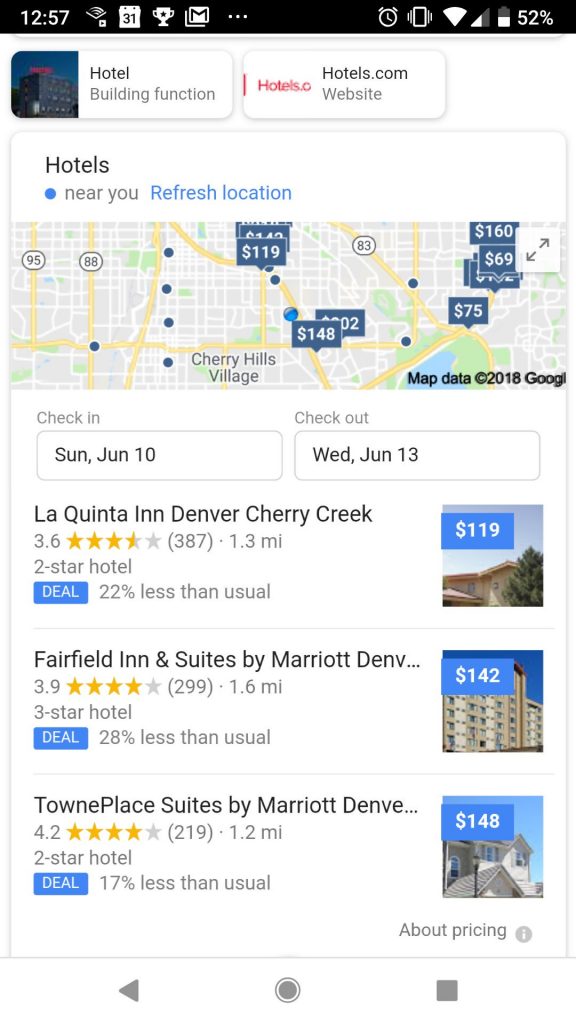In this photo, we see a smartphone screenshot displaying a hotel booking interface. At the very top, a black status bar spans across the screen, showing the battery level at 52% on the far right, with a Wi-Fi signal icon next to it. On the left, the time reads 12:57. Directly below this bar, there are two buttons: the left one labeled "Hotel" under the "Building Functions" category, and the right one labeled "Hotels.com" for navigating to the respective website.

The central part of the screen features a map marked with multiple hotels and their prices. Yellow roads, interwoven with smaller white roads, crisscross the map, while blue location dots indicate available hotels near the user's current position. There is also a refresh button for updating the location shown on the map.

Prices for the hotels are prominently displayed on the map, with offerings ranging from $69 to $160. Below the map, fields for entering check-in and check-out dates are visible. Further down, three specific hotels are listed in detail; two of them are rated as two-star hotels and one as a three-star hotel. Each listing includes various Google reviews and specifies the distance from the user's current location, providing a comprehensive snapshot of available accommodation options.